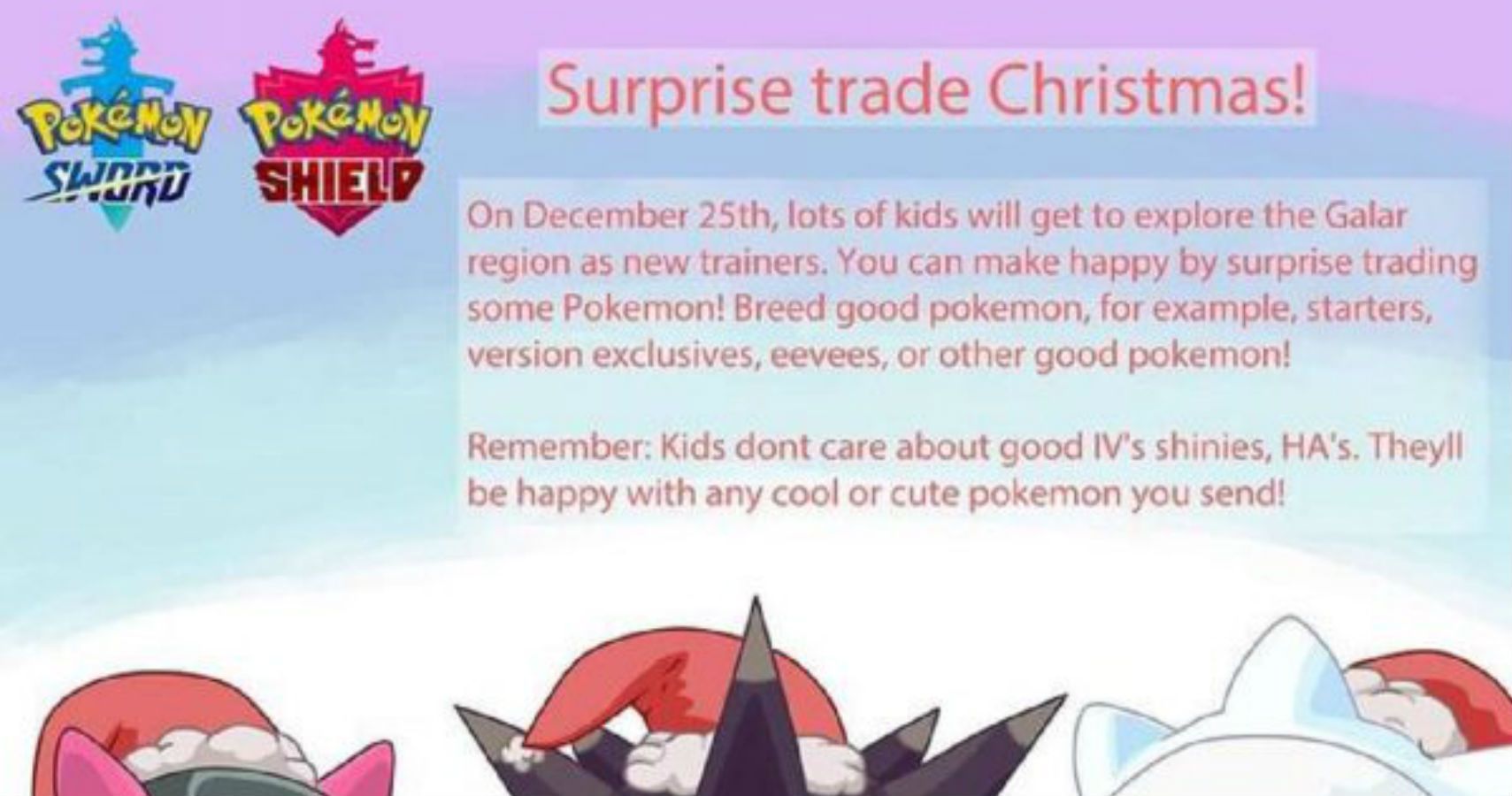This illustration showcases a rectangular image with text extending horizontally across the longer dimension. The scene captures the upper portions of three cartoon-like characters, arranged from left to right, all adorned with festive headgear. 

Starting from the left, we see the top of a character's head, revealing two pink ears protruding from a gray head. This character is wearing a red cap with white trim, reminiscent of a Christmas hat. 

To the right, the second character sports a similar red Christmas hat, complete with white trim and a white pom-pom. This character's head is adorned with five distinctively spiky points of hair or fur, colored in varying shades of gray, progressing from dark gray at the base to light gray at the tips.

In the far right corner, the third character's head is mostly obscured, leaving only the white top and cat-like white ears visible. This character also dons a red cap with white trim similar to the others.

Together, the trio creates a festive, cartoonish scene dominated by festive red and white headgear and the unique detailing of their ears and fur.